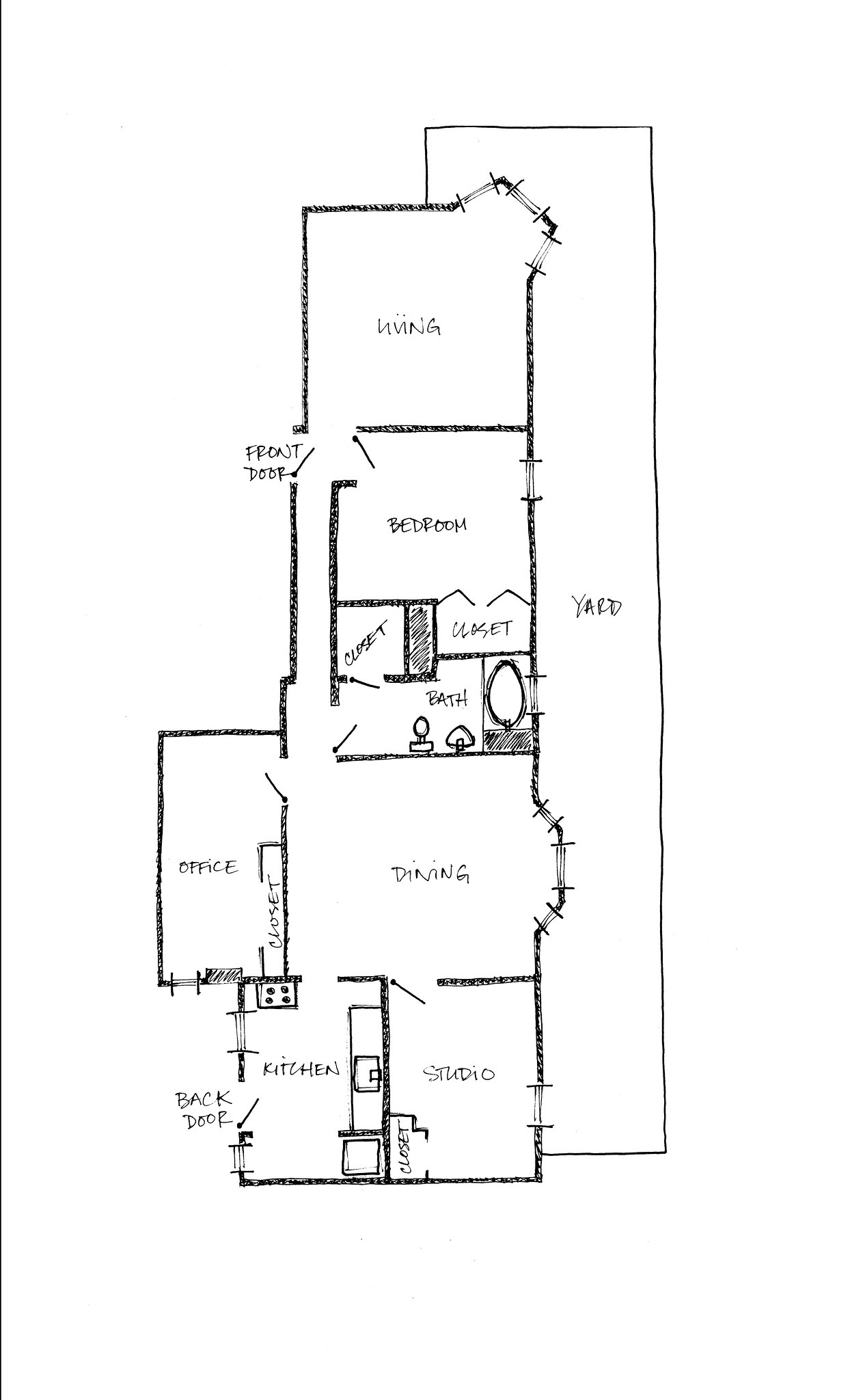This intricate, hand-drawn floor plan depicts a long, vertically oriented rectangular ranch house. The drawing is executed with precision, devoid of any underlying grid or graph paper, set against a pristine white background. 

Starting from the bottom of the plan, the layout begins with a kitchen adjacent to a studio, both leading into a spacious dining room. A small office extends off the main rectangle at the back, creating a slight protrusion but maintaining the overall compact shape. Moving upward, the house maintains its narrow form, featuring a bathroom and a closet. A long hallway runs along the left side of the house, connecting a series of rooms. A bedroom is located off this hallway, and further up is a living room with visible doors providing access.

The yard is situated on the right side of the house, but the main entrance is on the left. Upon entering through the front door, one's view is directed towards the bedroom door. To the immediate left is the living room. Continuing down the hallway, one encounters the bathroom, and further along, the dining room with the office protruding subtly from the main structure, followed by the kitchen and studio. The detailed and thoughtfully arranged floor plan captures the essence of a creatively designed but straightforward ranch house.